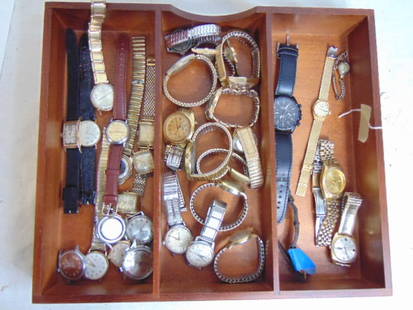This detailed image captures an open, three-compartment drawer, seemingly from a jewelry box, constructed from what appears to be maple wood, resting on a white countertop. The drawer hosts a diverse collection of approximately 40 analog watches for both men and women, showcasing an array of colors and materials. In the first compartment, one finds watches with black, gold, and brown leather bands, along with a pocket watch without a band. The middle compartment features watches predominantly with aluminum or steel bands, appearing silver with some gold accents, many of which lie on their sides, resembling gold bracelets. The final compartment contains a more eclectic mix, including a striking black watch with a matching black face and band, a watch with a blue-hued element at the bottom left, and various gold and silver watches of different designs. Notably, a piece of tape with attached string is visible on the side of the drawer, along with some blue tape inside, suggesting a lack of strict organizational scheme.